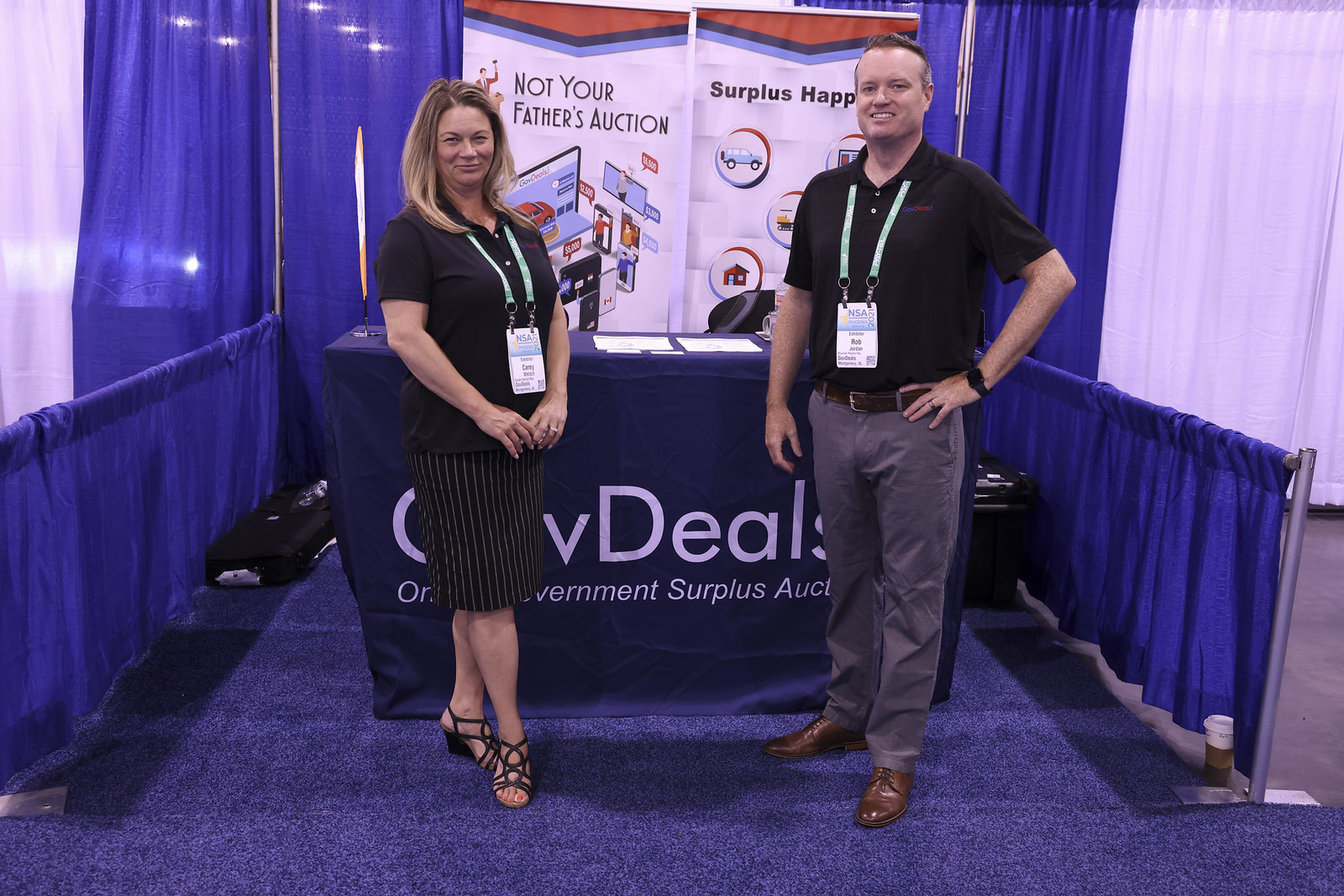In this photograph taken at a trade show, a man and a woman stand in front of a vendor booth adorned with deep purple and blue gauzy curtains on three sides, along with a matching blue rail draped in fabric at the bottom. The pair are positioned on a blue carpeted floor, smiling at the camera. Behind them is a table covered with a navy blue tablecloth, partially obscuring the white text which includes the words "DEALS" and "GOVERNMENT SURPLUS AUCTION." Two prominent banners feature the slogans "NOT YOUR FATHER'S AUCTION" and "SURPLUS."

The woman on the left has blonde hair and is dressed in a black short-sleeved top and a black and white skirt, complemented by black strappy high heels. On the right, the man wears a black collared shirt, gray pants, and brown dress shoes. Both individuals are sporting green lanyards around their necks, identifying them as representatives or employees of the company they're promoting.